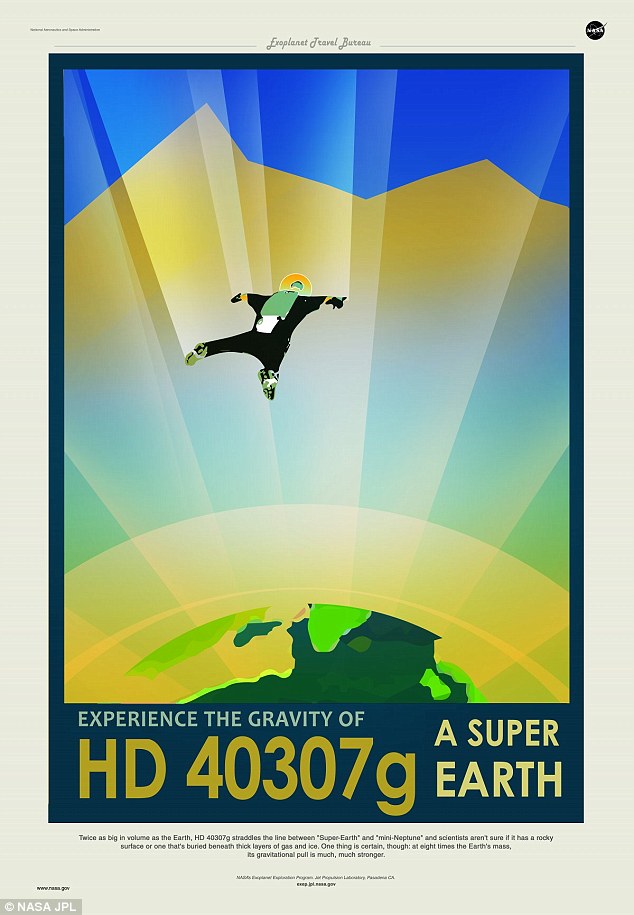This is a promotional illustration designed to attract attention to the Exoplanet Travel Bureau. It features a striking, computer-generated graphic art style. The main focus is a skydiver, clad in a black outfit with a green parachute, free-falling toward an artistically rendered planet. The planet, a green and yellow globe with a lime green hue, is depicted amid glowing beams of light radiating outward, creating a luminous yellow aura. The skydiver appears to be experiencing the stronger gravitational pull of this celestial body. The backdrop comprises a blue and yellow gradient, with the planet positioned near the lower section, giving the impression of the vast expanse of space.

Encasing the image is a detailed border: a white border surrounding a slimmer black one, with the NASA logo prominently featured in the upper right-hand corner. There is an evident promotion by NASA's Jet Propulsion Laboratory (NASA JPL), as noted by the copyright in the bottom left-hand corner. The text, set in varied fonts and colors for emphasis, boldly states: "Experience the Gravity of HD 40307 G, a Super-Earth." Additional information printed at the top identifies this as material from the Exoplanet Travel Bureau. The description emphasizes that HD 40307 G is a super-Earth, twice the volume of our planet, potentially with either a rocky surface or one covered in thick layers of gas and ice, and it highlights the planet's significantly stronger gravitational pull due to its eight times greater mass.